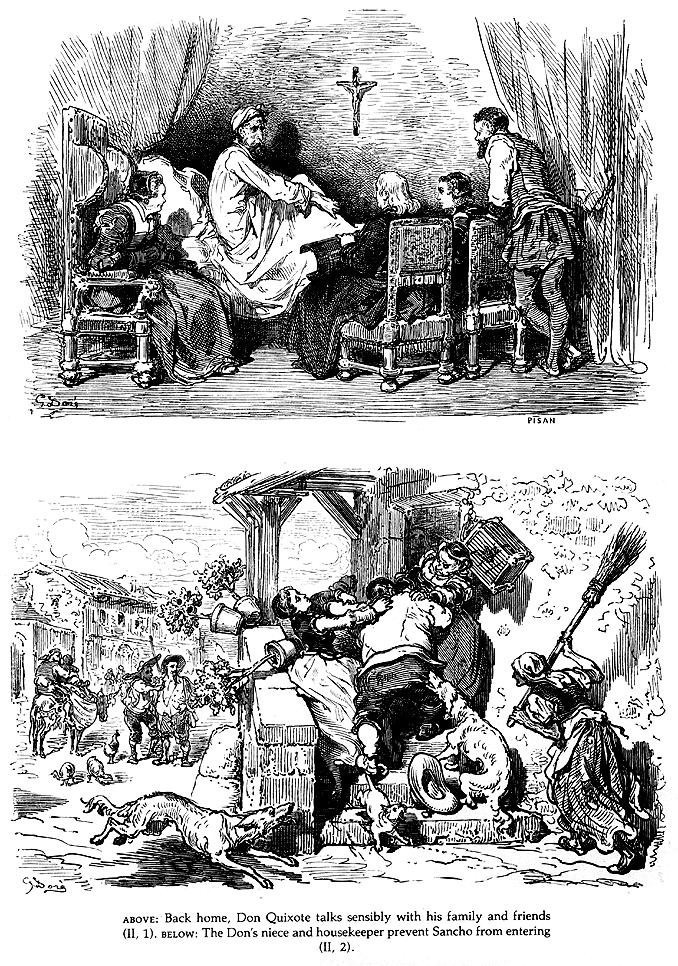This image features two detailed black ink sketches of scenes from Don Quixote, rendered with intricate line work. The top illustration depicts Don Quixote standing beside a chair, engaging in conversation with his family and friends who are seated around a table. The setting is dominated by a crucifix on the wall behind them, adding a solemn tone to the gathering. A notable detail is an old woman seated to Don Quixote’s right, who looks at him with eager anticipation.

The lower illustration captures a chaotic outdoor scene. Don Quixote’s housekeeper, wielding a broom, along with several dogs and other townsfolk, attempts to prevent Sancho from entering an edifice. Multiple people are involved in this struggle, with outstretched arms clashing and potted plants being knocked over in the commotion. Amidst the hectic scene, a small dog runs around, contributing to the sense of disorder. In the background, a village street and additional onlookers can be seen, observing the ruckus. 

Text below the illustrations reads, "Above, back home Don Quixote talks sensibly with his family and friends. Below, Don's niece and housekeeper prevent Sancho from entering."